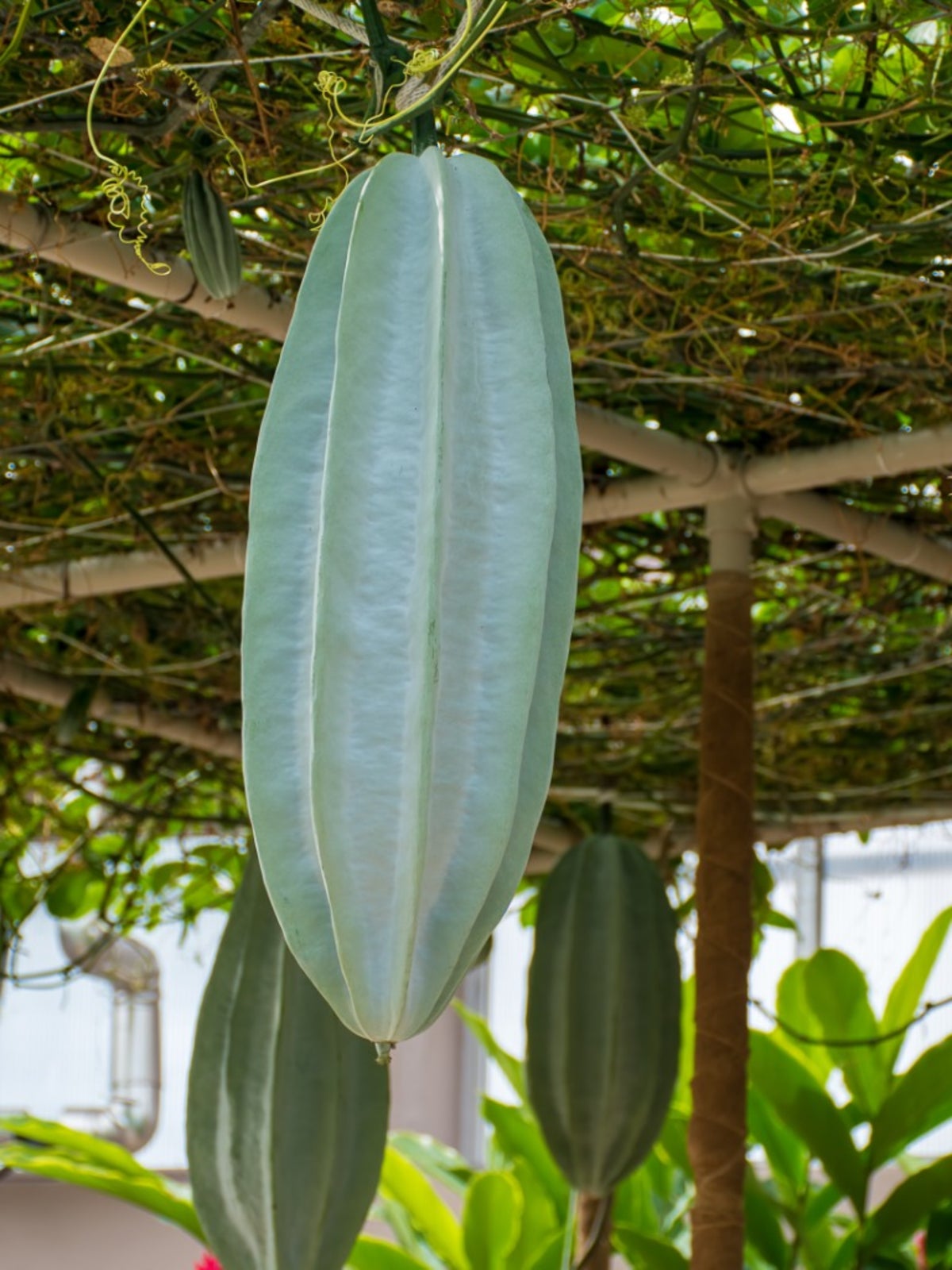In a green nursery setting, the image features a makeshift trellis structure made of steel poles and fencing supporting a network of green vines and thatch. Hanging from this trellis are elongated, cylindrical green pods, measuring up to 24 inches long and 6 to 8 inches thick. These pods, which resemble large cucumbers or melons, are pale green with sharp ridges running their length. The scene includes multiple pods, with three prominent ones in the foreground and additional smaller and similarly shaped pods in the background. The structure also features an iron gutter for runoff, and the lush green setting emphasizes the thriving plant growth.